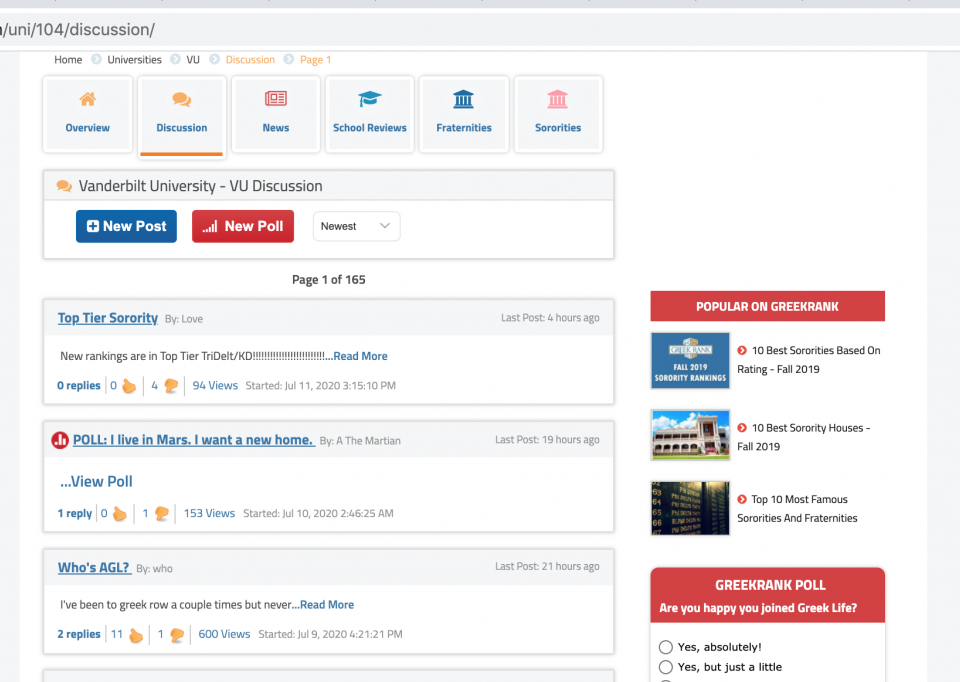Category: Websites

The image appears to be a screenshot of a discussion forum focused on universities. The top part of the screen is partially cut off, but visible text indicates it belongs to a thread titled "Uni 104 Discussion," with more text likely preceding it. Directly below this title, a navigation bar lists the following breadcrumb links: Home, Universities, VU, Discussion, and Page 1. 

Below the navigation bar, there are several clickable square tabs: Overview, Discussion, News, School Reviews, Fraternities, and Sororities, with the "Discussion" tab highlighted. 

The section under the discussion tab features an area titled "Vanderbilt University, VU, Discussion," accompanied by options to create a "New Post" (blue button with white text) or a "New Poll" (red button with white text). There is also a drop-down menu currently set to "Newest," with other sorting options not visible.

Listed discussions include:
1. **Topic: "Top Tier Sorority by Love"**
   - **New Rankings are in: Top Tier Tri Delt KD!!!**
   - "Read more" link in blue text.
   - Statistics: Zero replies, four thumbs down, 94 views
   - Initiated: July 11, 2020, at 3:15:10 PM.

2. **Poll: "I live on Mars, I want a new home"**
   - Author: A. the Martian
   - "View poll" link available.
   - Statistics: One reply, one thumbs down, 153 views

3. **Discussion: "Who is AGL?"**
   - "I've been to Greek Row a few times but have never..."
   - Statistics: Eleven thumbs up, one thumbs down.